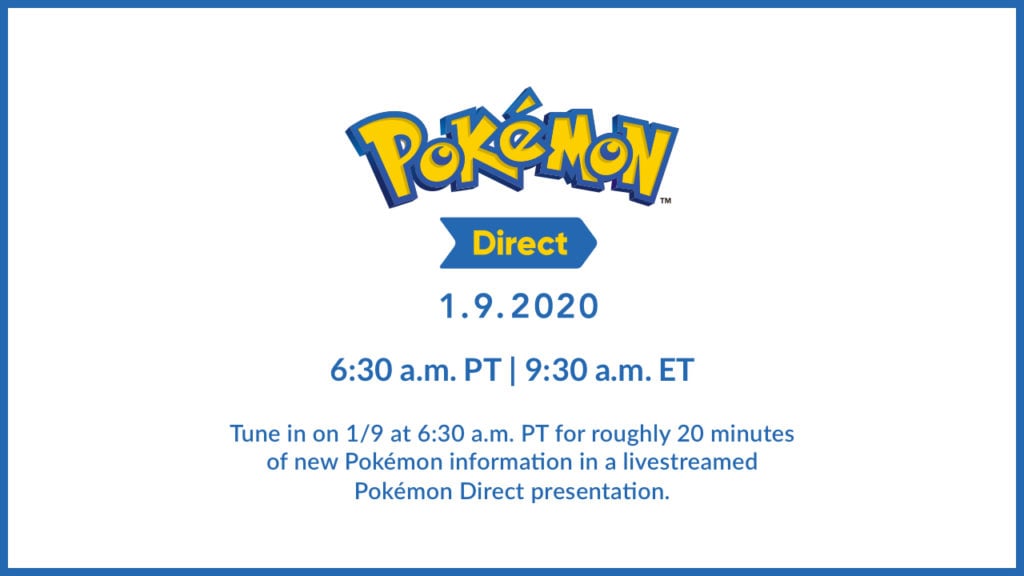The image features a white background framed with a blue border. Dominating the center is the traditional Pokémon logo, prominently displayed in yellow with a trademark symbol to its right. Below the logo, a thick blue arrow points to the right and contains the word "Direct" in bold yellow text. 

The image appears to be an announcement for a Pokémon Direct event, scheduled for January 9, 2020. The date is formatted as "1-9-2020" and is highlighted next to specific times - 6:30 AM Pacific Time and 9:30 AM Eastern Time. Underneath these details, additional text invites viewers to "tune in on 1/9 at 6:30 AM PT for roughly 20 minutes of new Pokémon information and a live stream Pokémon Direct presentation."

The design layout is predominantly blue and yellow, with "Direct" in yellow to match the Pokémon logo, which also features a black trademark symbol. The text describing the event is smaller and spans across multiple lines for clarity. The Pokémon logo artistically curves slightly, with "Poké" rising diagonally and "mon" trailing downward. There are no visual markers indicating that this image is sourced from a specific device, suggesting it might be a copy of an advertisement or announcement poster.